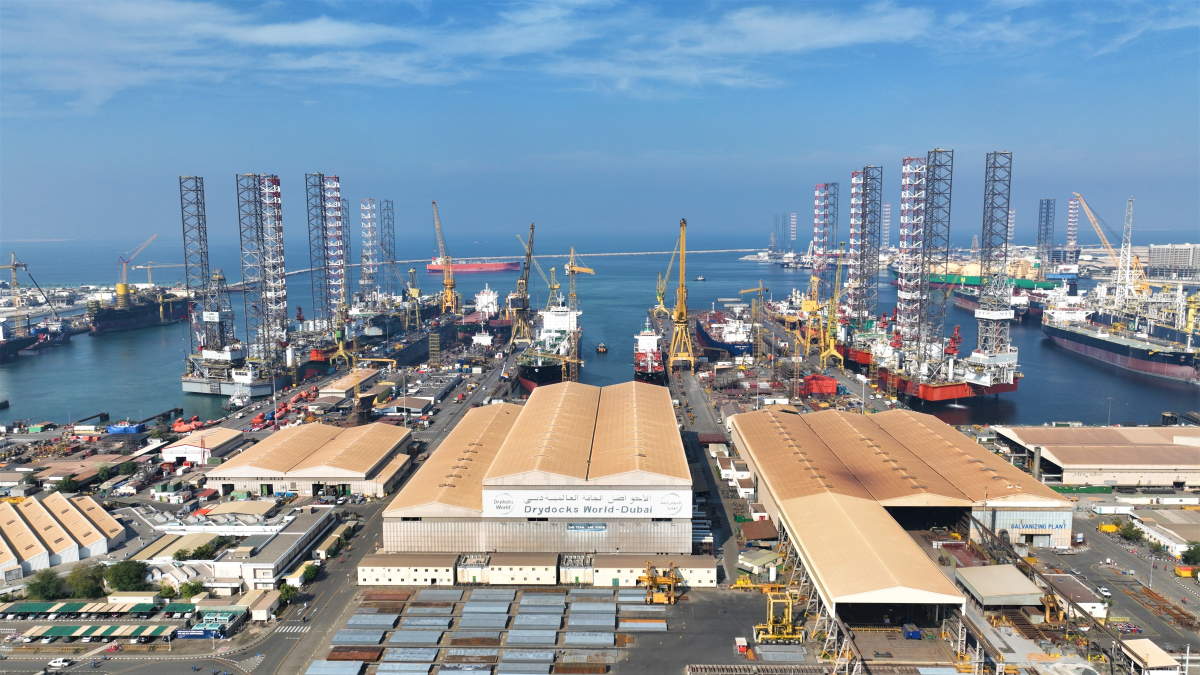This is an aerial, somewhat overhead view of a bustling shipyard, likely in Dubai, as suggested by a sign indicating "Dry Docks World of Dubai." The image captures a large open water area dotted with numerous cargo ships and boats, all aligned with towering metal scaffoldings and rigs protruding from some of the vessels. Surrounding the water are concrete roadways and docks lined with shipping containers in the process of being loaded or unloaded. Prominently, yellow cranes with hooks dangle towards the ground, standing ready to assist in the heavy lifting. In the background, you can glimpse the blue expanse of the ocean meeting a sky scattered with white clouds. The port area also features large covered building structures, possibly for storage or manufacturing, along with smaller sheds and parking areas filled with vehicles, including trucks and semi-trailer trucks. The diverse array of colors, including red, white, blue, black, green, brown, and yellow, brings vibrancy to this industrial seaport scene, likely photographed from a high vantage point, showcasing the intricate and busy operations of maritime logistics.